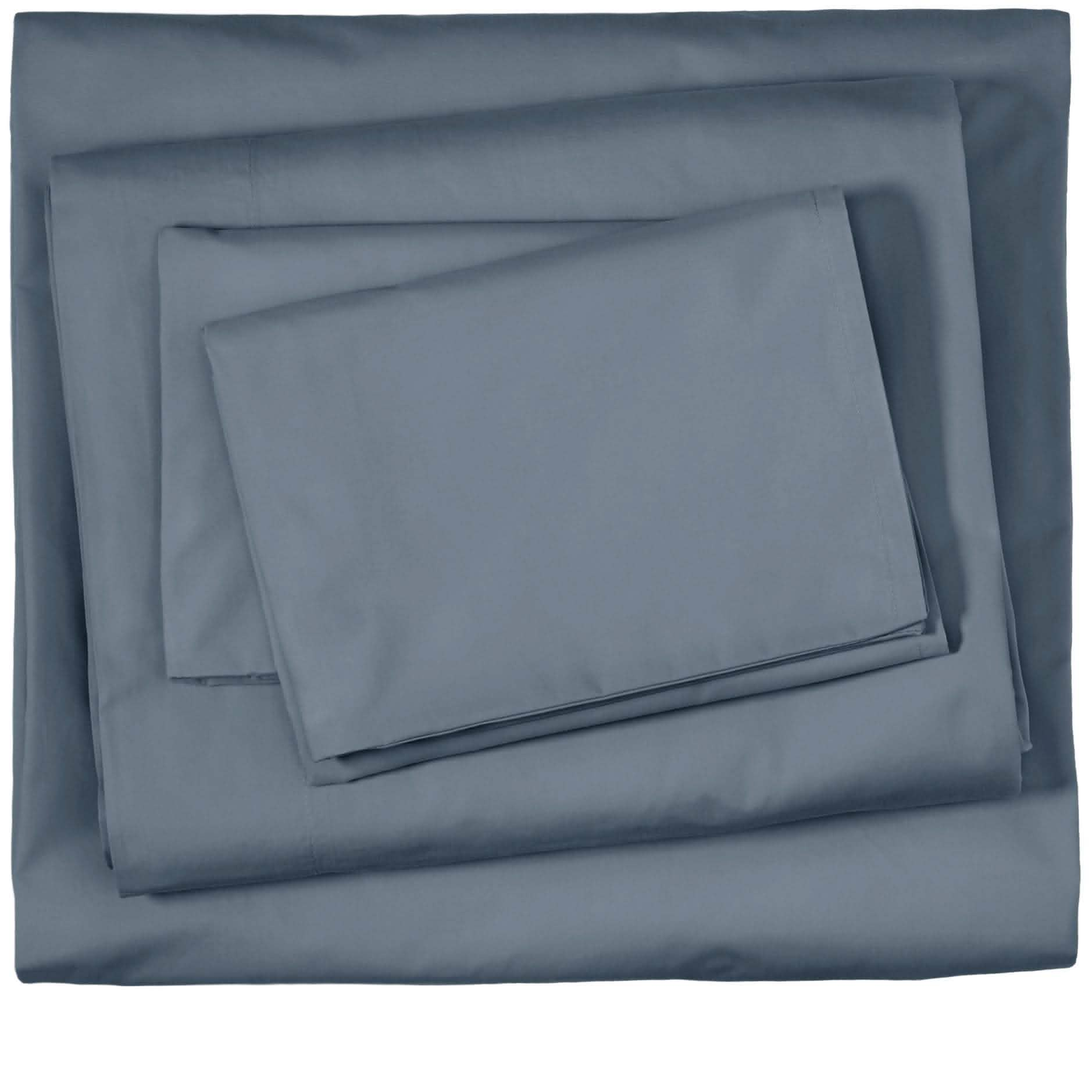This is a detailed image of a neatly folded, full set of bed sheets likely designed for a king-size bed. The sheets are a dark, steely gray color, leaning towards black, with no patterns—just plain, solid color. Composed of what appears to be cotton material, the sheets give off an impression of fine weaving and high quality. The set includes a large sheet at the bottom, a slightly smaller sheet atop it, and two smaller pieces, likely pillowcases, stacked on top. The photo, taken from an eagle's eye view, captures the sheets perfectly aligned and flat against a white backdrop, emphasizing their clean, minimalist design. The well-lit image exudes a sense of simplicity and elegance, resembling professional product photography often seen in online catalogs.